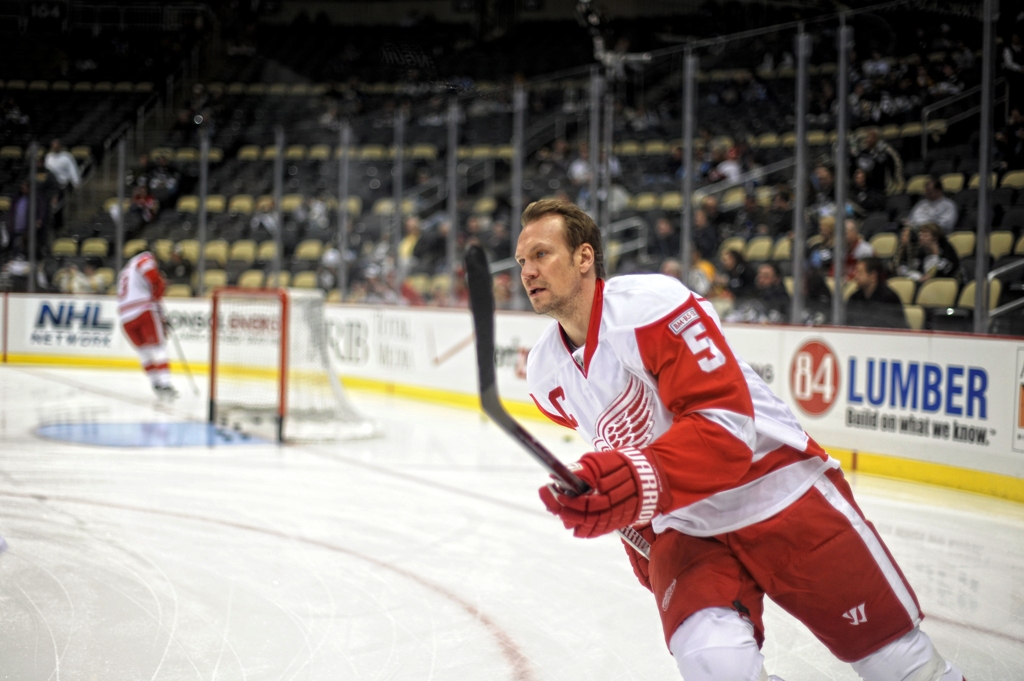In the image, two Detroit Red Wings hockey players are seen practicing on the ice rink before a game. The player on the right is prominently featured, holding his hockey stick with both hands and wearing a complete Red Wings uniform, which includes a white long-sleeved jersey with red sleeves, red padded shorts, white knee pads, and red gloves. Notably, he is without a helmet. The jersey bears a red wing logo on the front, and the number five is visible on his shoulder. He appears to be in his 30s or 40s with light brown hair.

In the blurred background, another player, also without a helmet, is noticeable near the hockey net, wearing the same Red Wings uniform. Between the two players stands the goal, which is currently unguarded. The background reveals a few fans in the stands, glass panels for protection, and various banners and logos, including those for NHL, Verizon, and 84 Lumber. The overall setting captures the pre-game preparation atmosphere on the ice rink.